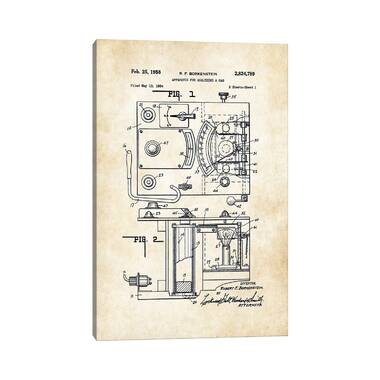The image depicts an aged, speckled parchment with a white and tan texture, suggesting historical significance. The centerpiece is a detailed drawing divided into two labeled figures: Figure 1 and Figure 2. Figure 1, depicted in the upper section, resembles a blueprint, possibly of a garden layout, featuring small circular elements and a rounded arch-like structure. Figure 2, located in the lower section, appears more mechanical or industrial, suggesting elements of water or machinery, hinting at a workspace environment.

Intricate text surrounds the image, with a notable date inscribed as February 25th, 1958. Additional annotations and numerical details adorn the top right-hand corner, while other textual elements are present at both the top and bottom of the parchment. A signature, discreetly placed in the bottom right-hand corner, adds a personal touch, possibly indicating the original creator or an authenticating mark. Overall, while the image contains many details, its distant perspective makes it challenging to discern the full extent of its content and purpose.